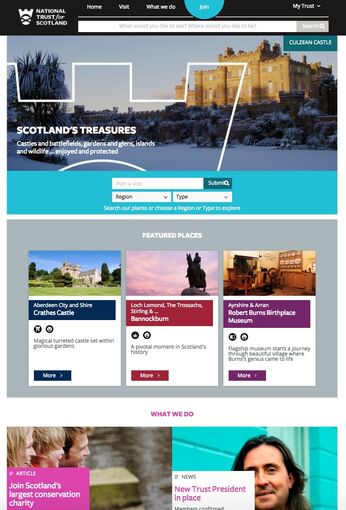The image appears to be a shrunken screenshot of a website, likely for the National Trust for Scotland. The header features a black background with white text, including a logo that depicts a crown and a figure, accompanied by the text "National Trust for Scotland." 

In the top navigation area, various menu options are displayed in white text: "Home," "Visit," and "What We Do." Adjacent to these, there's a half-visible blue button or circle that says "Join" in white text. On the far right, there is a "My Trust" option with a dropdown arrow, and beneath this navigation bar is a search bar with grey text that is illegible due to the image's resolution.

Prominently featured is a stunning photograph of a light-tan Scottish castle against a baby blue sky, with snow-covered ground. The text "Scotland's treasures" appears in white over this image, along with additional, smaller text that is unreadable.

Below this main image, there seems to be an area dedicated to searching for flights or other options. This is followed by a section labeled "Featured Places," accompanied by an image of a statue inside what looks like a pub.

At the bottom of the image, there is a scene of a family enjoying a show, their expressions filled with laughter and joy. This section includes text inviting viewers to "Join Scotland's largest conservation charity." To the right, there is a photo of a man looking directly at the camera with the caption "New Trust President" in black text on a white background located at the bottom left of the image. 

Overall, the website layout is designed to entice visitors with vibrant images of Scotland's landmarks and provide various navigational options to explore more about the National Trust for Scotland.